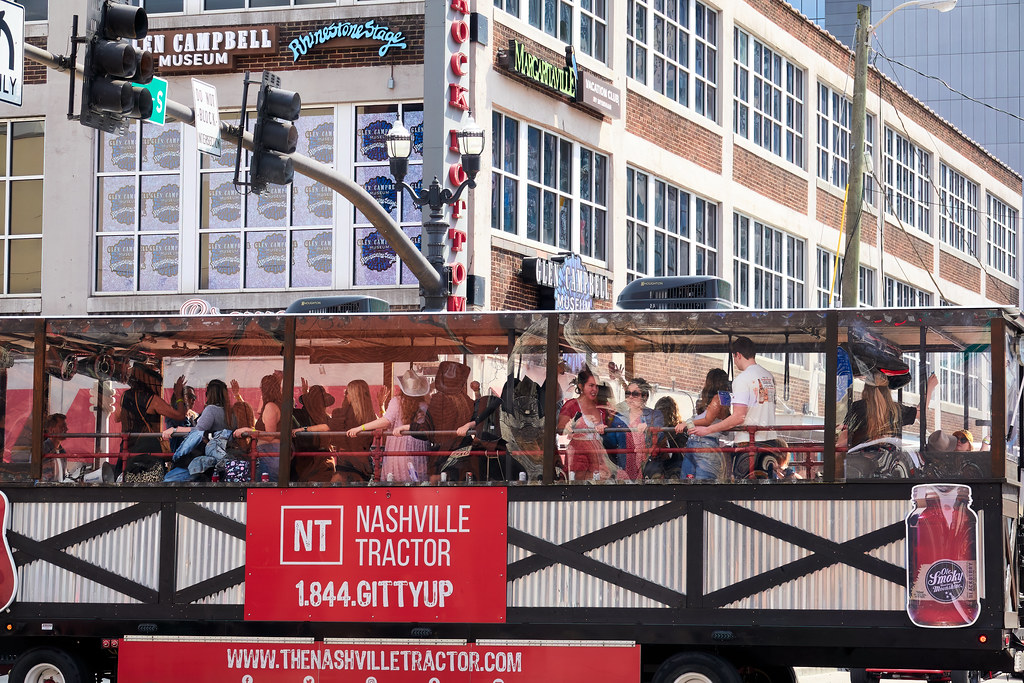This is a color photograph taken outdoors in a bustling city street, likely Nashville, Tennessee. The image showcases a unique vehicle resembling a farm tractor outfitted for a city tour or party, often called a "party tractor." Prominently featured on the side of the trailer is an orange sign reading "NT Nashville Tractor 1-844-GITTYUP" and another sign below that says "www.thenashviltractor.com." The vehicle has corrugated steel half walls with black X-like barn door designs as well as sections made of glass or plastic.

A diverse group of people is seen either sitting or standing along the gray rail of the tractor. From right to left, the people include a blonde man wearing a large hat, a white man in a white t-shirt with a green and orange graphic, a white woman in jeans and a light blue shirt, another white woman with sunglasses, a white woman in a red shirt, two people in cowboy hats (one black, one white), and other individuals including a blonde woman taking a photo and a woman in a white tank top holding onto the rail.

In the background, the vibrant cityscape includes a multi-story brick building with white window frames. Prominent signage for the "Glen Campbell Museum" and its "Rhinestone Stage" can be seen, along with a green "Margaritaville" sign. A vertical sign for the "Rock Bottom" restaurant is also visible. The sky in the background is clear and blue, adding to the lively atmosphere of this daytime city scene.